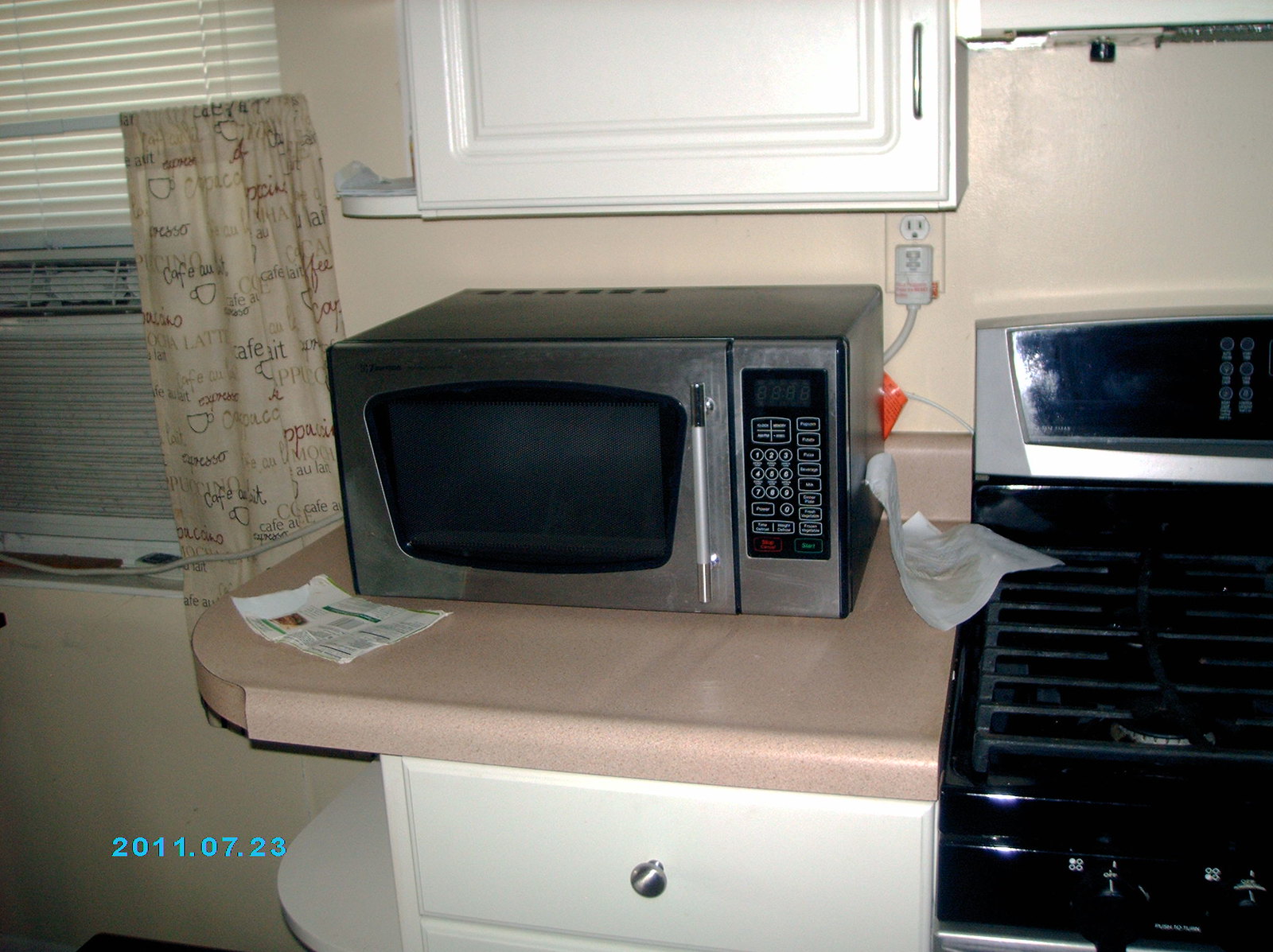The image captures a vintage kitchen, prominently featuring a stainless steel microwave positioned centrally on a cream-colored countertop with rounded edges. The microwave, likely from the mid to late 2000s, boasts a black control panel with white lettering, including distinctive red and green buttons at the bottom. Above the microwave is a partially visible white cabinet with silver handles, and below it begins a series of white drawers. Adjacent to the microwave, a black gas stove with cast iron burners shares the countertop space. To the left of the countertop, an air conditioning unit is installed in a window with blinds at the top and open café-style curtains adorned with coffee cup motifs. In the bottom left corner of the image, a date stamp in blue font reads "2011.07.23," marking the photograph as taken 13 years ago, which aligns with the slightly outdated design of the kitchen. A restaurant-style napkin with writing is present on the countertop, adding to the room's detailed yet nostalgic ambiance.